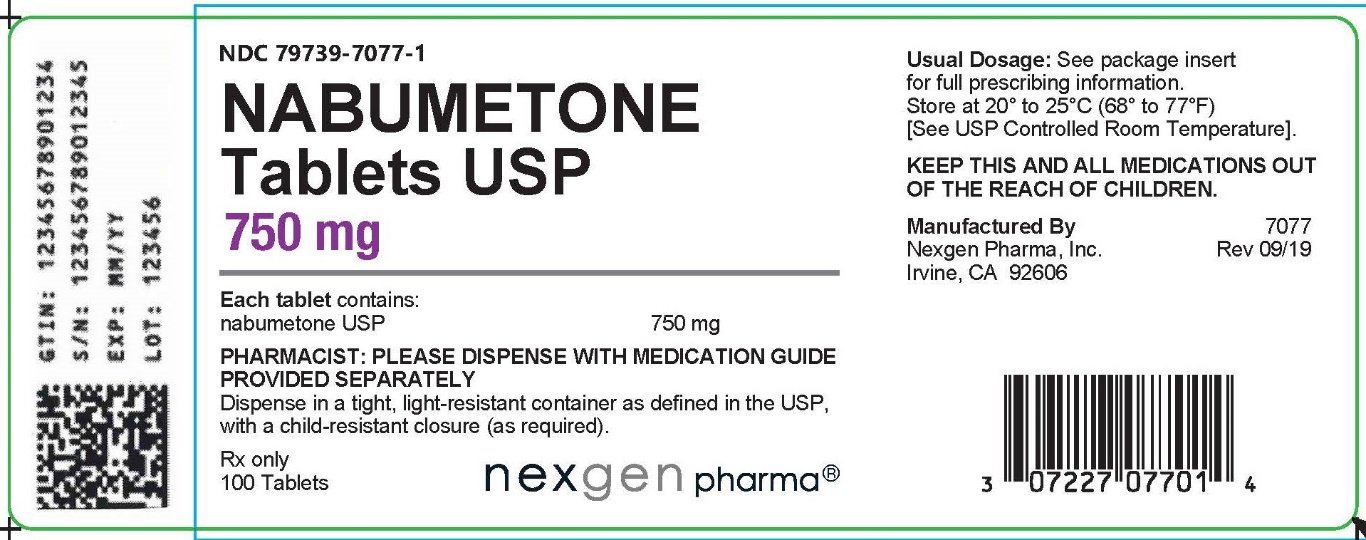### Detailed Caption for Packaging Design Image of Nambumetone Tablets

This image showcases the packaging design for Nambumetone 750 mg tablets, developed by Next-Gen Pharma, Inc. The packaging is clearly marked "Rx-only," indicating that these tablets are prescription-only medications. The container is specified as tight and light-resistant to protect the tablets and maintain their efficacy as per USP (United States Pharmacopeia) standards. Precise storage instructions are provided, recommending a controlled room temperature of 20°C to 25°C (68°F to 77°F). 

Additional details include the manufacturing information, with the product being crafted by Next-Gen Pharma, Inc. under the lot number 7077, and a verification location in California with the zip code 92606. The packaging date is noted as Rev. 09-19. The image also features a barcode with the number 30722707014 for tracking and identification.

Important safety information is prominently displayed, advising users to keep the medication and all other drugs out of the reach of children to prevent accidental ingestion or misuse. The design elements and regulatory information emphasize the manufacturer's commitment to safety, compliance, and quality.

In summary, the image depicts a professionally designed pharmaceutical packaging that contains all necessary information to ensure proper handling, storage, and usage of the Nambumetone 750 mg tablets.